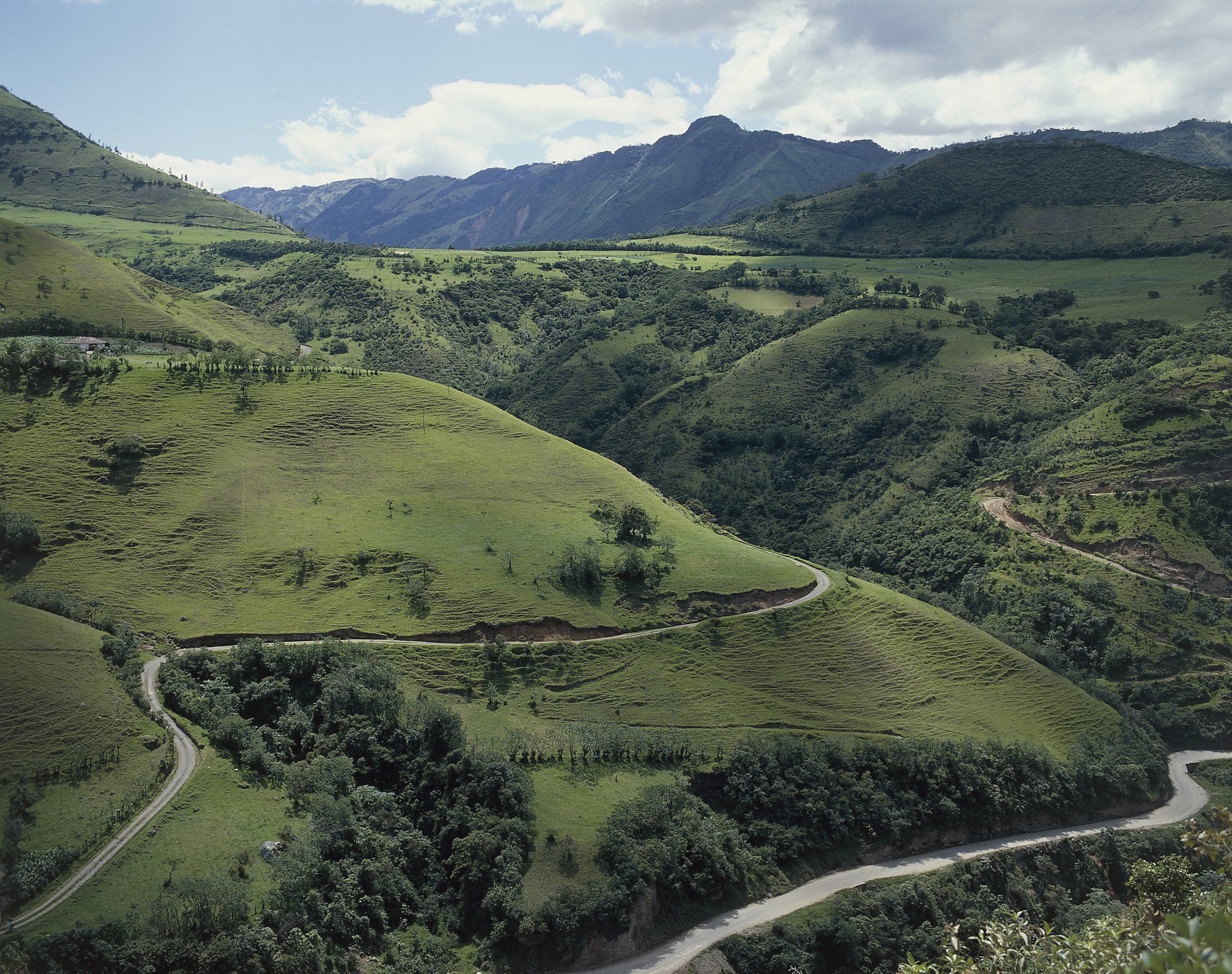The color photograph, captured from an aerial perspective, showcases a lush, hilly landscape draped in vibrant greens. The gentle, rolling hills are sprinkled with patches of darker green trees, creating a striking contrast amid the swathes of lighter green grass. Two winding roads meander through these verdant hills; one road starts at the bottom left, elegantly curving in an S shape before vanishing around a central hill, while the more prominent path cuts through the bottom center, veering towards the bottom right and reappearing further up in the distance. Beyond the hills, a formidable mountain range, tinged with dark blue hues, stands against the horizon. The backdrop is crowned by a light blue sky, partially veiled by white clouds on the top right, adding a sense of depth to the scene. The entire setting is bathed in a soft, hazy sunlight, emphasizing the natural beauty captured through photographic realism.